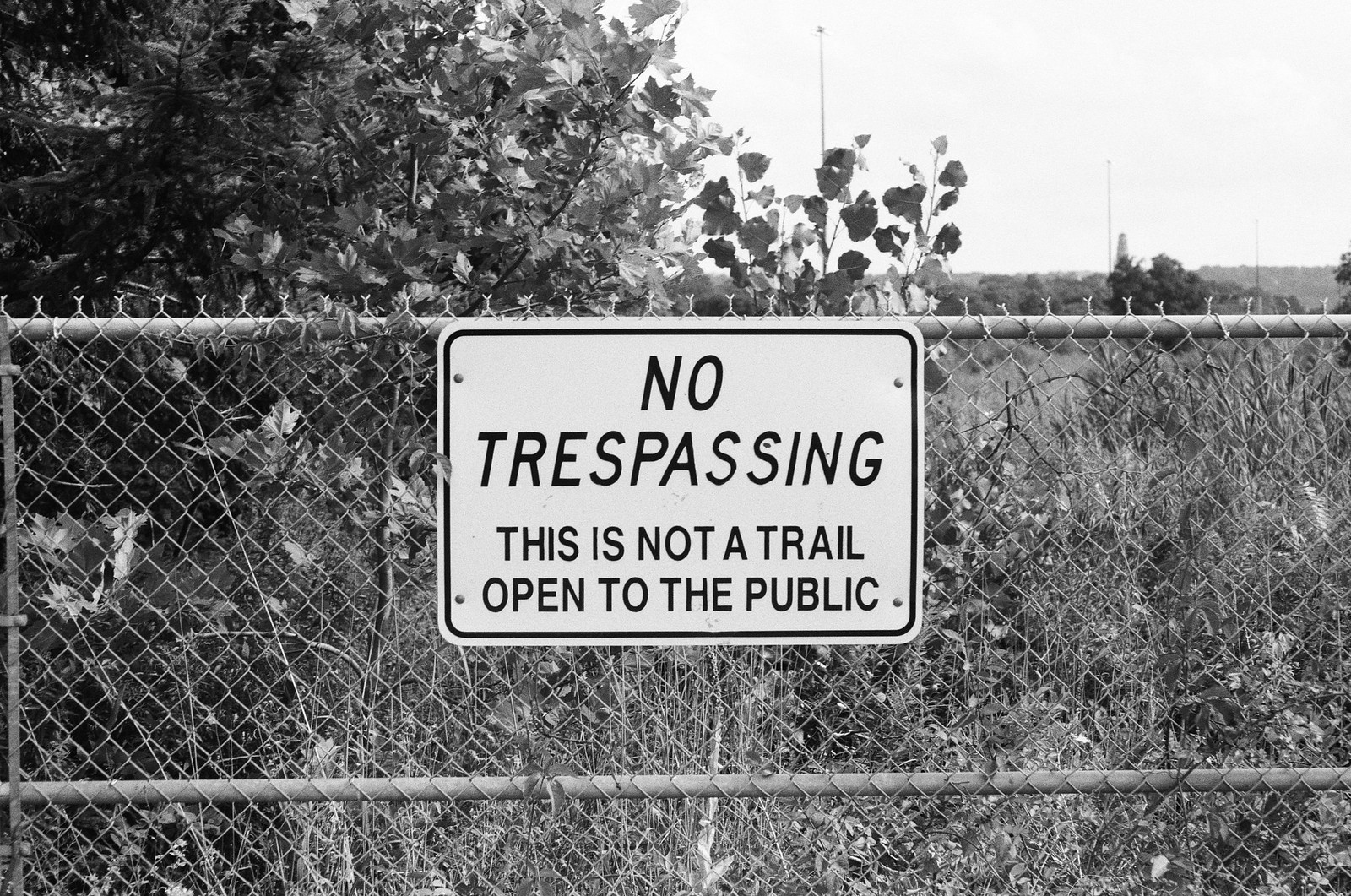This black and white photograph, taken outdoors, captures a detailed scene dominated by an aluminum fence adorned with a prominent rectangular sign. The sign is white with a smaller black rectangle within it, boldly stating "No Trespassing" at the top, and below, in smaller letters, "This is not a trail, open to the public." Behind the fence stretches a landscape filled with an array of trees, shrubs, and bushes, extending into a distant field. The sky above appears overcast, hinting at cloudy weather. Farther back, subtle traces of what might be a road are hinted at by poles, potentially light posts, that can be seen in the hazy background.